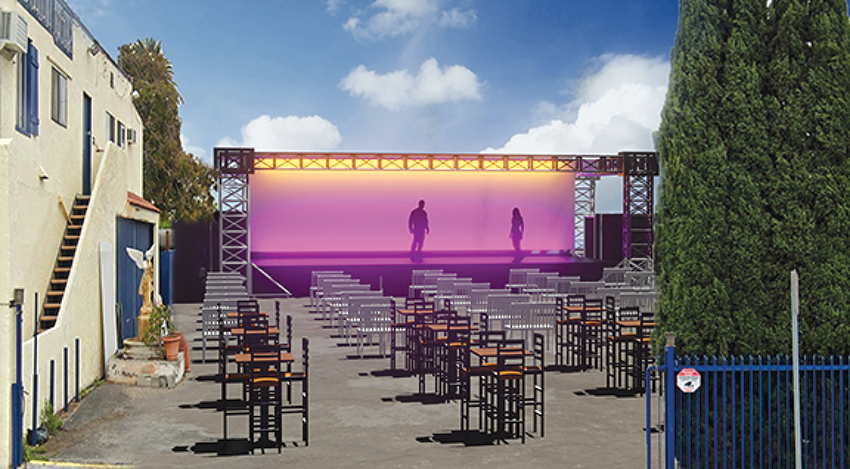The photograph, taken outside during the day, features a prominent purple-lit stage with a man and a woman silhouetted against the bright yellow lights. The sky is a clear blue with puffy white clouds dispersed across the center and right. To the bottom right, there’s a small blue fence adorned with an ambiguous white sticker with red at the top. The right side of the image is dominated by a large green tree, its height extending beyond the frame. In the foreground, rows of seats are aligned, with the closer seats appearing white or chrome, while farther back, wooden-topped tables with black chairs are arranged. Leftward stands a light cream or yellowish building with blue doors and window shutters, and a narrow staircase leading to an upper level. The ground below is a stark gray, resembling concrete. The scene appears devoid of a crowd, with an air of abandonment around the empty seating area and the open blue gate leading to the theater setup.